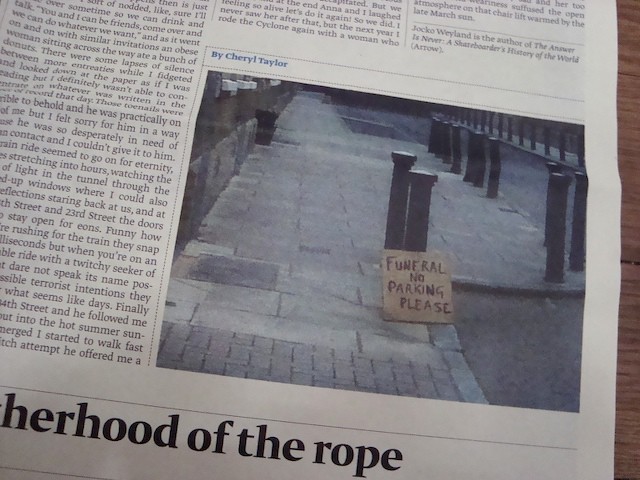This image is a detailed photograph of a section of a newspaper displayed on a dark wooden surface, visible as a narrow sliver on the right-hand side. Dominating the newspaper is a central photograph, showing a paved gray-bricked sidewalk lined with several small black metal poles. Leaning against one of these poles is a piece of cardboard with handwritten black lettering that reads, "Funeral, No Parking Please." Above the photograph, the caption in blue font reads "by Cheryl Taylor." Below the photograph, in thick black font, is the headline "Her Hood of the Rope." The newspaper itself is white with various columns of black text, though the majority of the article text is cut off and not fully visible within the image.